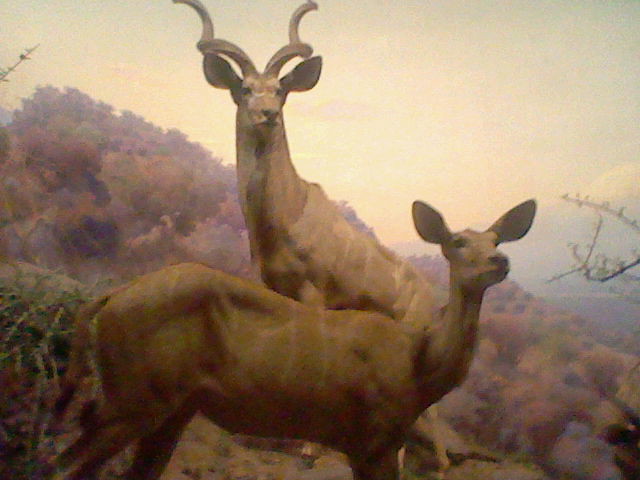This image appears to be a photograph of a painting or an illustration from a textbook, showcasing two deer—a buck with curled antlers and a doe without antlers—standing side by side in a colorful autumn forest. The background features a vibrant tapestry of fall leaves against a mountainous horizon, with some clouds visible but mostly sunny. The realistic portrayal of the deer and their surroundings, with hills and trees in the backdrop, suggests it may belong to a natural history museum exhibit or a biology textbook. The lifelike yet artistic depiction of the scene lends a majestic quality to the deer, both of whom are gazing away from the camera, adding an element of serenity to the image.